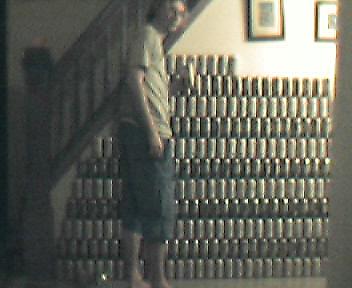The image is a slightly wider than tall, grainy and somewhat gloomy photograph, suggesting it could be from an older device. The primary subject is a man standing in front of a meticulously stacked tower of beer cans, approximately eight cans high and twenty wide, going up to his chest. He's wearing a gray or whitish t-shirt and knee-length dark gray or khaki shorts, barefoot, and is positioned near a wooden staircase on the upper left. His head is turned towards the camera, likely looking at the person who took the photo, and he appears to be holding a can, about to add it to the structure. The backdrop includes an off-white wall with two black-framed images above the beer cans, though the content of these frames is unclear. The ambient light source shines from the upper right, casting the left side into deeper shadow. The overall small and dark nature of the image underscores its possible age.